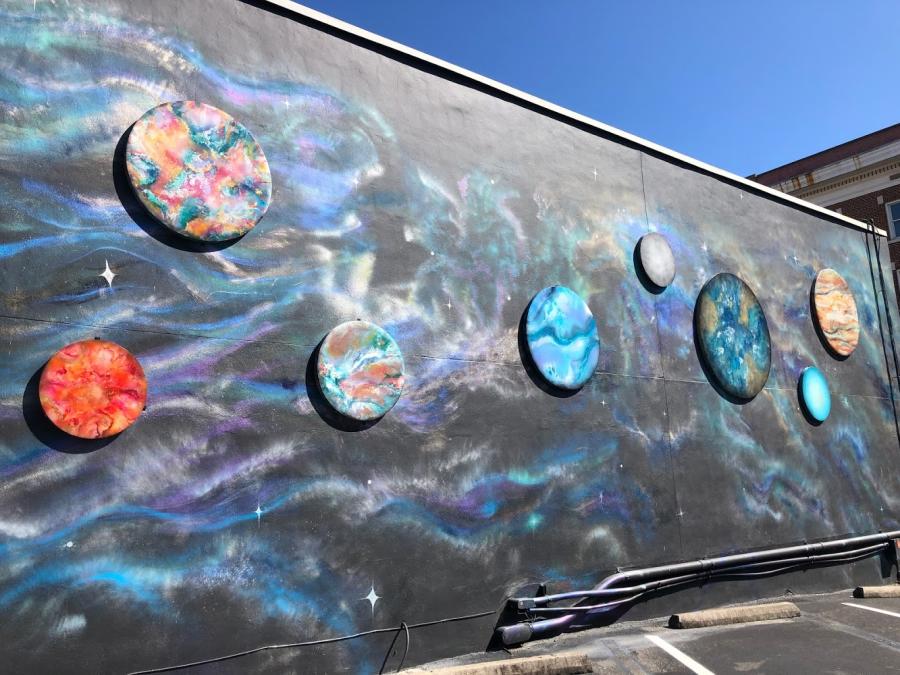This photo captures an outdoor scene of a mural painted on the side of a building, situated near a parking lot with visible concrete parking stops. The mural, likely representing the Milky Way, features eight circular discs, each painted to resemble different planets. These discs vary in size and color, including representations of Earth, the Moon, and Jupiter among others. The background of the mural is predominantly black, adorned with wispy streaks of blue, purple, and white, mimicking a galaxy or nebula. Pipes and conduits emerge from the bottom of the wall, adding an additional layer of detail to the scene. The photograph, taken in daytime, also captures a clear blue sky in the upper right corner, indicating the sun is shining on the mural.